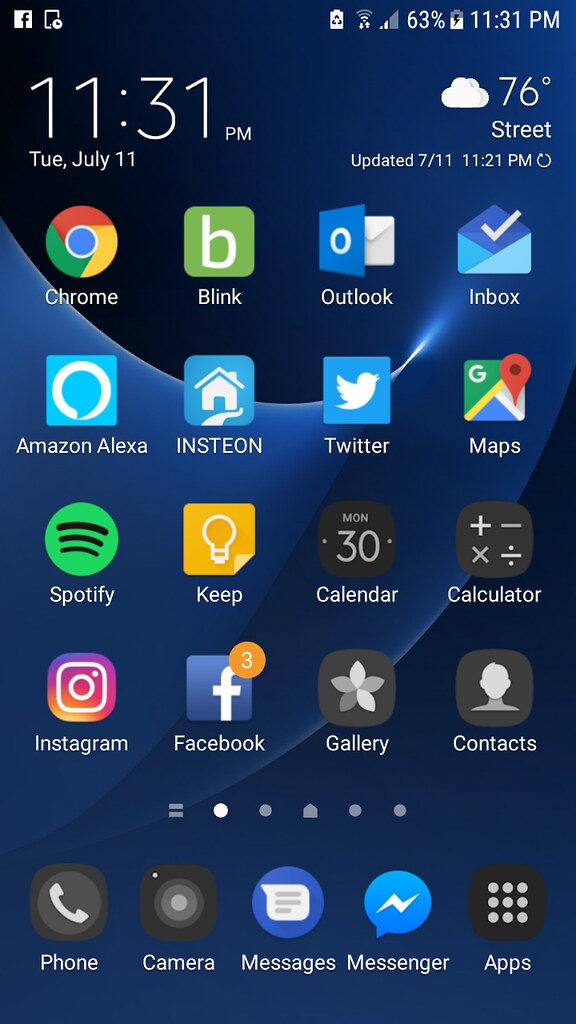This screenshot captures the home screen of an Android smartphone. The screen is densely populated with various app icons, indicating a user who actively engages with a variety of applications. The status bar at the top displays the current time and date on the left side, while the right side shows the weather information.

The central portion of the screen is filled with numerous app icons including, but not limited to, Chrome, Blink, Outlook (Inbox), Maps, Twitter, Insteon, Amazon Alexa, Spotify, Keep, Calendar, Calculator, Contacts, Gallery, Facebook, and Instagram. Below this array of apps, there are several navigation buttons.

At the very bottom of the screen, quick access icons are displayed, providing easy reach to essential functions such as Phone, Camera, Messages, Messenger, and a shortcut to all other apps.

The background of the home screen has a blue theme with a gradient resembling ocean waves, featuring different shades from blue to black, accented with hints of white light.

Considering the design and style of the app icons, this screenshot seems to date back a few years, reflecting an earlier version of the Android operating system.